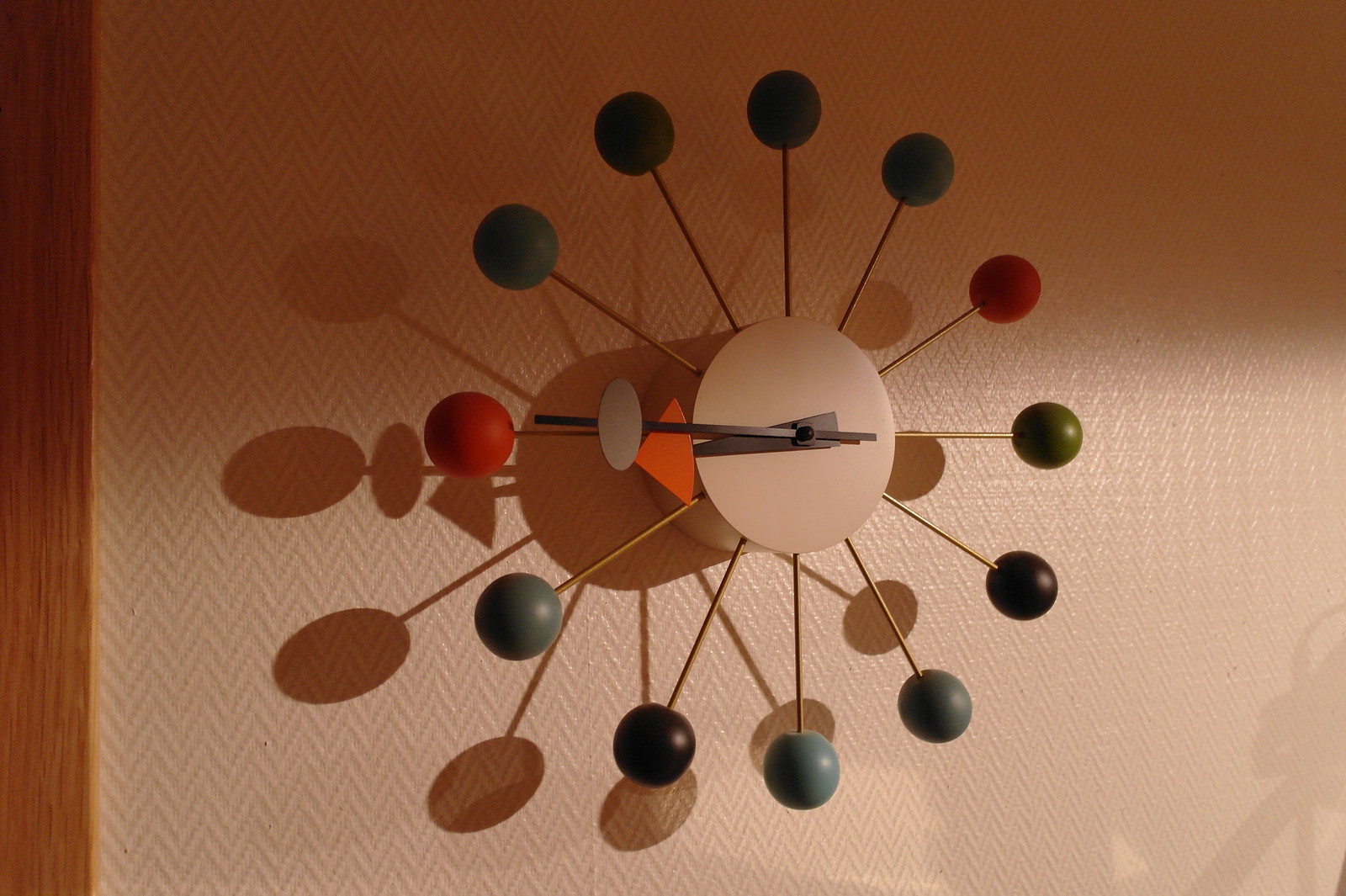In the image, there is a modern, artistic clock mounted on a wall adorned with cream-colored, zigzag-patterned wallpaper. At the center of the clock is a pale pink circle from which multiple gold rods radiate outwards like spokes. Each rod is tipped with a colored ball in varying hues: red, olive green, black, blue, and gray. The clock's hands are made of dark chocolate brown metal; the hour hand features an orange triangular tip, while the minute hand is distinguished by an oblong, oval-shaped piece near its end. The clock design includes more than the traditional twelve spokes, adding to its contemporary aesthetic. The shadow of the clock is cast on the wall, complementing the overall visual interest of the piece.